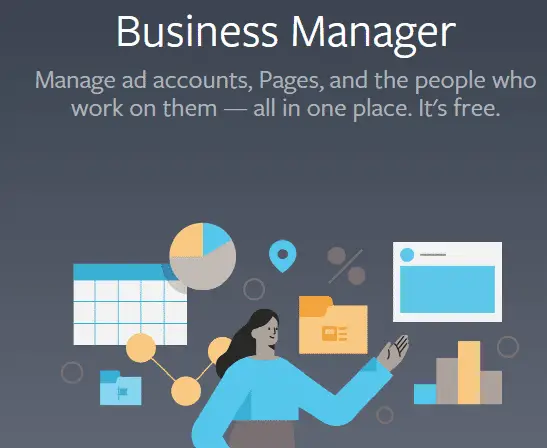This image appears to be an advertisement for a business management tool. It features a minimalistic design set against a dark gray background. At the top, white text prominently displays the phrase "Business Manager." Below this title, additional text explains the tool’s functionality with the message: "Manage ad accounts, pages, and the people who work on them - all in one place. It's free."

Central to the image is a graphic showcasing various elements associated with business management. These include icons and illustrations such as a calendar, pie chart, graphs, folders, locations, percentages, a bar graph, and a prototype of a social media page, effectively highlighting the diverse capabilities of the tool.

On the bottom right, there's a cartoon depiction of a woman with long black hair, wearing a blue shirt and brown bottoms. She is gesturing to the right, drawing attention to the surrounding cartoon graphics. The overall composition effectively conveys the comprehensive features of the business management tool in a visually engaging manner.